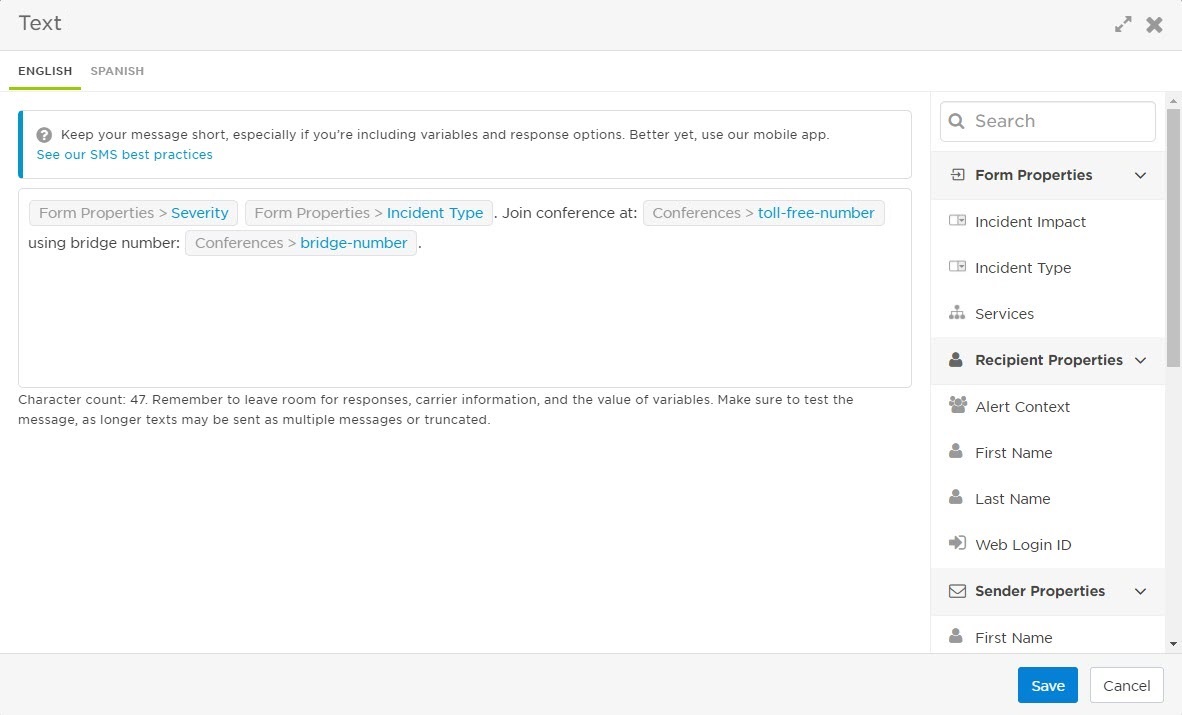A screenshot of a messaging application interface is depicted. At the top of the interface, there is a long bar with the word "Text" located in the upper-left corner. In the upper-right corner, there are two diagonally aligned arrows: one pointing up and the other pointing down, alongside an "X" button. Below the word "Text," "English" is underlined in green, with "Spanish" as the alternative option.

A message header is urging users to "keep your message short especially if you're including variables and response options. Better yet, use our mobile app." Following this, in blue text, a clickable link states "See our SMS best practices."

Next, there is a section labeled "From Properties," featuring an arrow pointing to the right and the word "Severity." Subsequent sections include "Incident Type," "Join Conference At," and "Conferences," all with clickable options in blue text. A subsection names a "Toll-Free Number" and another subsection with the labels "Using Bridge Number" and "Conference," with the bridge number highlighted in blue text on the right.

To the far right, there is a search bar. Below this, several dropdown menus are visible: "Form Properties," which includes options for "Incident Impact," "Incident Type," and "Services." Another section labeled "Recipient Properties" presents choices like "Alert Context," "First Name," "Last Name," and "Web Login ID." Finally, there is a section labeled "Sender Properties," which is accompanied by an envelope icon, and an option to click on "First Name."

Overall, the interface appears well-organized, providing users with multiple sections to tailor their message properties and recipient details efficiently.